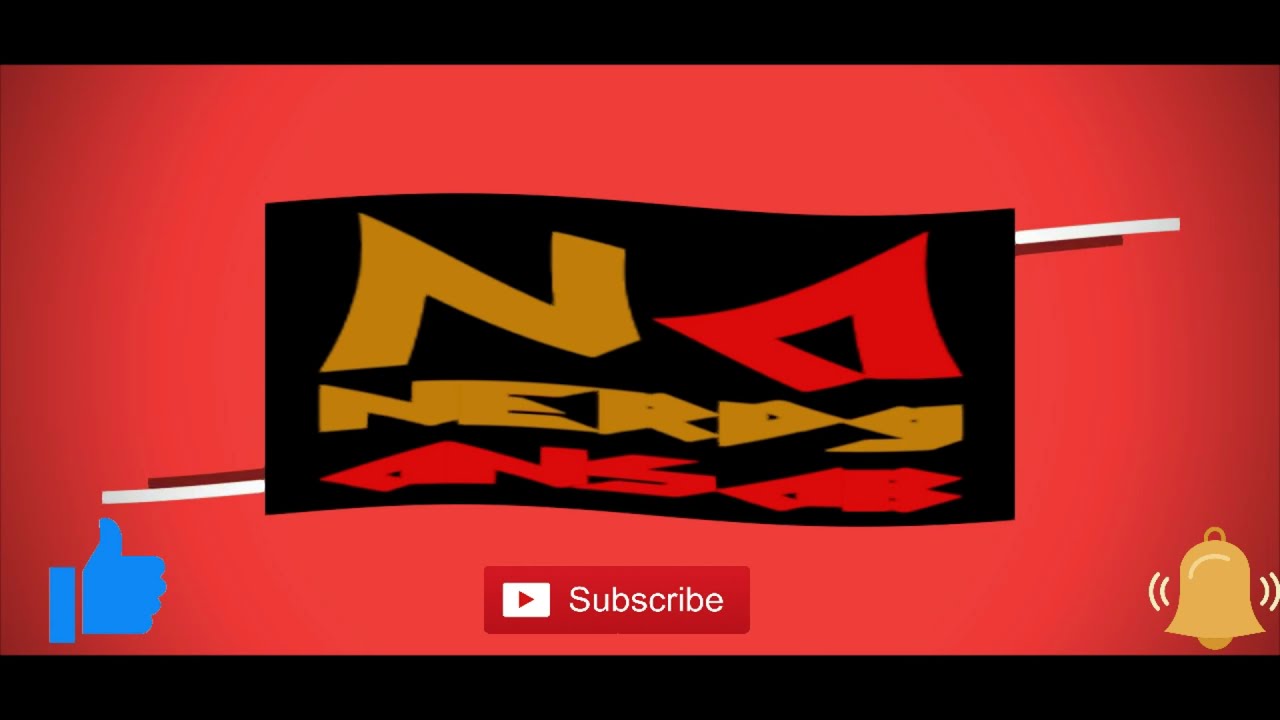This image, likely a graphical design for a YouTube advertisement, features a vivid red background with a gradient effect that transitions from light at the center to dark at the edges. Central to the design is a wavy black rectangle resembling a flag, adorned with intricate gold and red text. At the top of the flag is a prominent gold letter "N," followed by what appears to be the word "NERDY" in bold, stylized letters. Below this, more text in red is visible but difficult to discern clearly. The flag is accentuated by white lines extending from its lower left, bottom, and right upper corners, adding a dynamic visual element.

On the lower part of the image, signature YouTube interface elements are present: a blue thumbs-up button on the left, a central red "Subscribe" button featuring a white play icon, and a gold bell icon on the right, emitting lines that indicate it is ringing or vibrating. The overall design is modern and digital, with a touch of artistic flair reminiscent of skater graffiti, suggesting an edgy and appealing aesthetic.